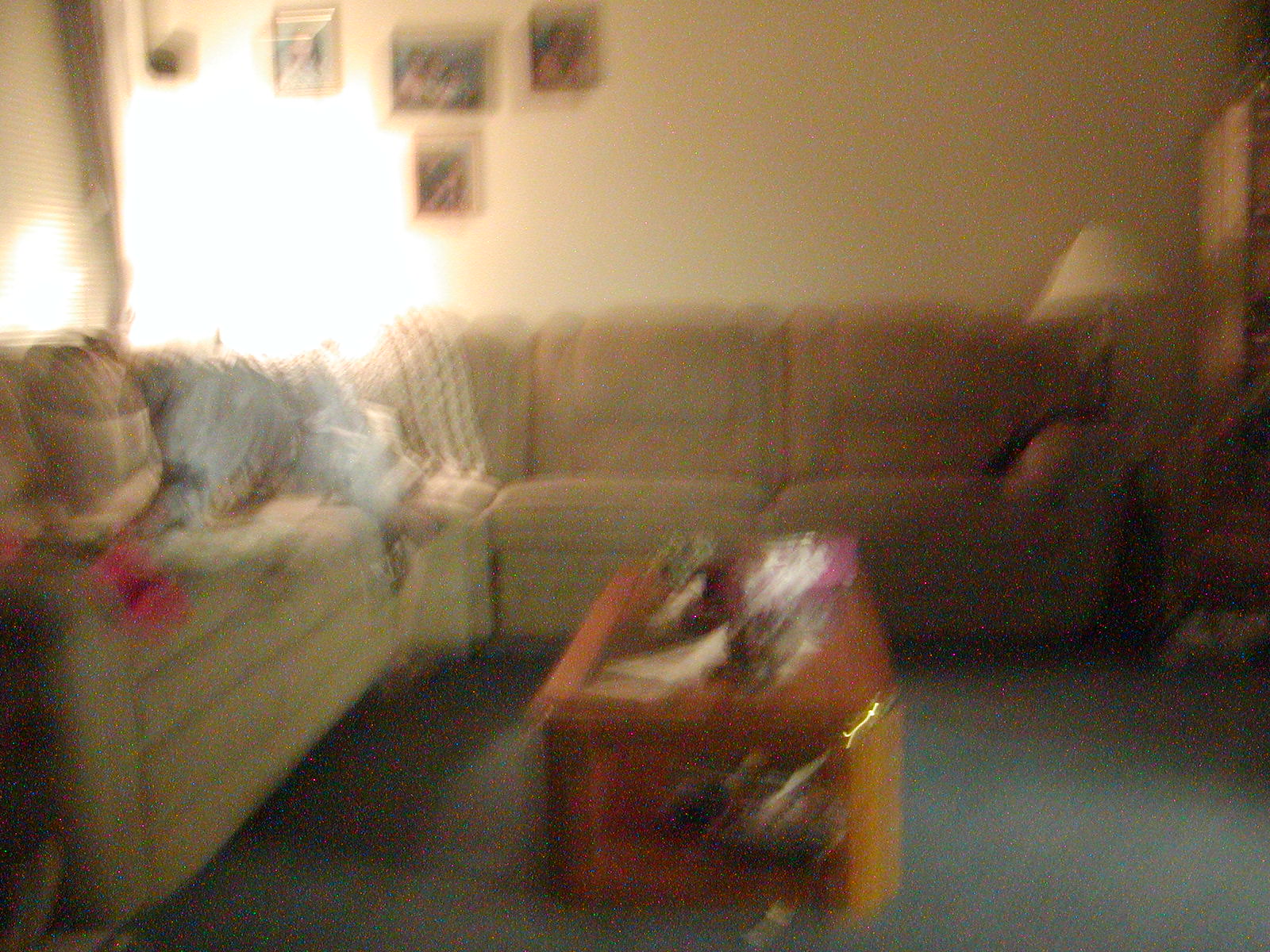This color snapshot depicts an indoor living room scene, captured with poor quality and out of focus, likely due to camera movement. The room is bathed in tungsten lighting, complemented by a bright light source situated in the upper left quadrant along the wall. Surrounding this light are small framed pictures that add a touch of personal decor.

Dominating the lower left quadrant and extending towards the center is a light brown or tan L-shaped sectional couch, cluttered with various objects—possibly pillows, blankets, or clothing—particularly concentrated beneath the light source. In the center of the room stands a coffee table, scattered with assorted items, adding to the lived-in feel of the space.

On the right side of the image, a bookshelf extends into view, accompanied by a standing lamp that provides additional illumination. The overall scene is tinged with a yellow hue, likely due to the tungsten lighting, which casts a warm glow over the entire setting. Despite the photograph's lack of clarity, the details suggest a cozy and personalized living area.